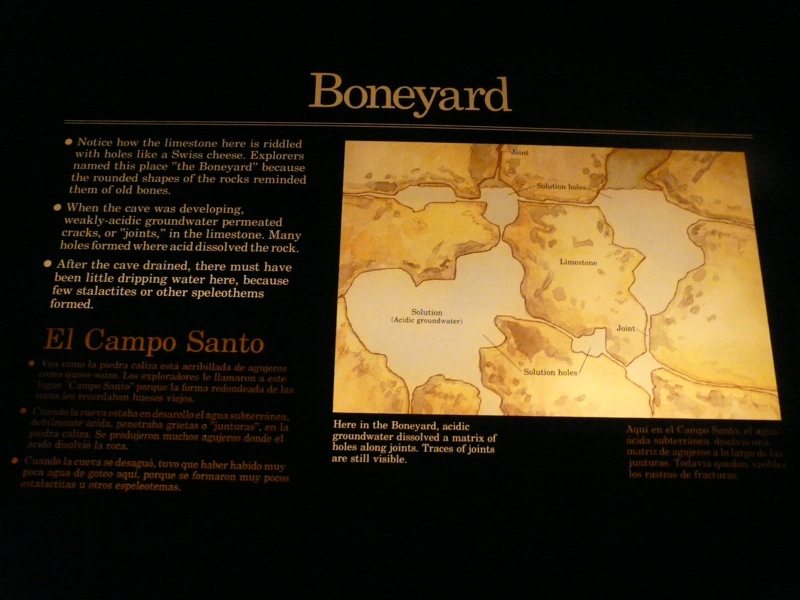The image is of a museum display with a black background. At the top of the display, in bold yellow letters, it says "Boneyard." To the right, there is a geological map with labels such as "limestone," "solution holes," "solution," and "acidic groundwater," depicted in various shades of brown. The map illustrates the landmasses and their positions, highlighting the impact of acidic groundwater dissolving a matrix of holes along joints, with traces of these joints still visible.

On the left side of the display, there is a section of text in light brown color, accompanied by three bullet points. The first bullet point reads: "Notice how the limestone here is riddled with holes like Swiss cheese.” This points out that explorers named the area "Boneyard" because the rounded shapes of the rocks resemble old bones. Below these bullet points, a paragraph explains the geological features, with the header noting "El Campo Santo" in red text. This descriptive and informative layout provides visitors with a comprehensive understanding of the Boneyard’s unique geological landscape.